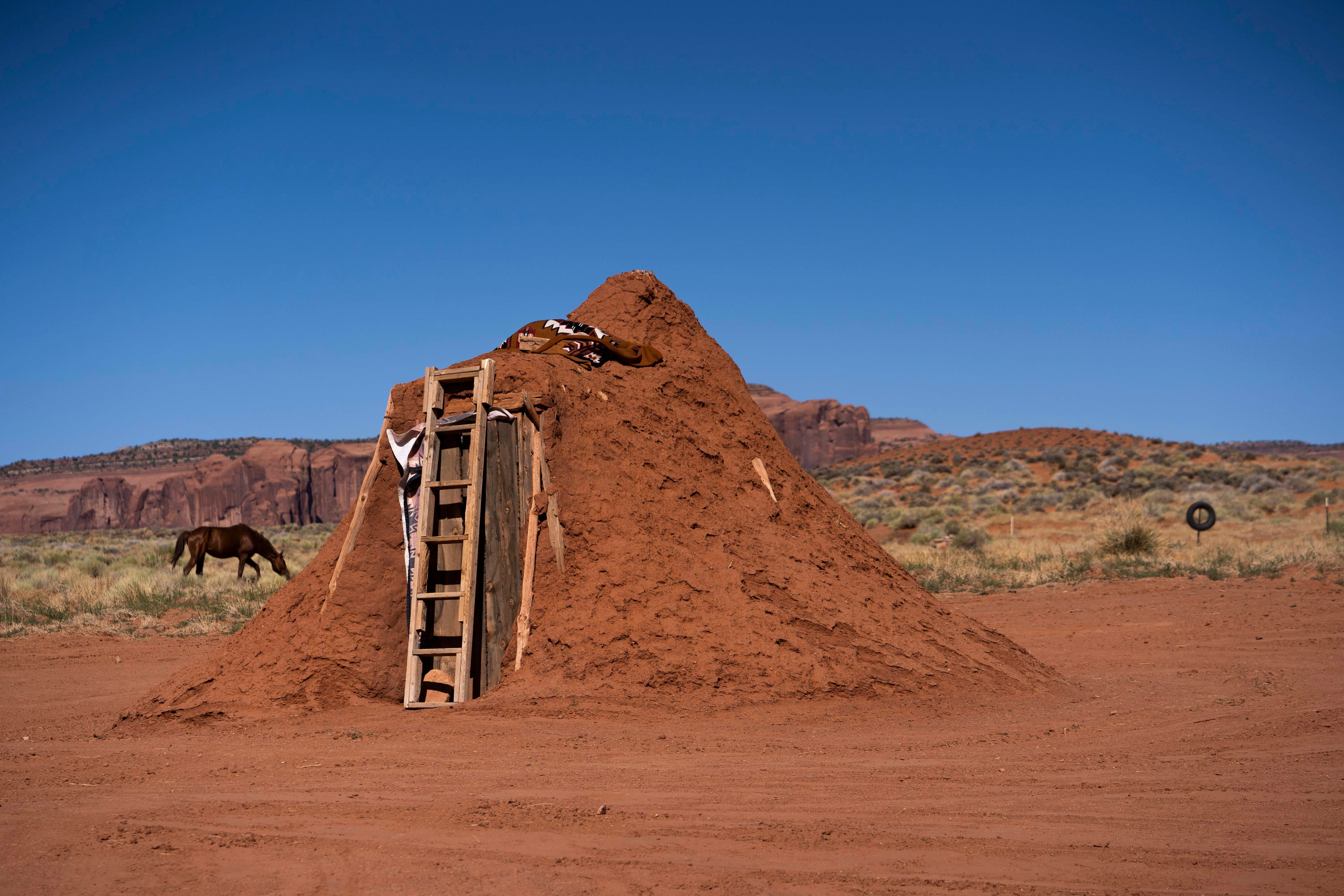This captivating image, evocative of an arid desert expanse reminiscent of regions such as Arizona or New Mexico, features a strikingly clear, bright blue sky devoid of clouds. The foreground is dominated by a rustic, mound-like structure composed primarily of dirt or mud, with a ladder leaning against it. This ladder appears to provide access to the roof of the structure, hinting at possible habitation. Adding to this intrigue is a small wooden door nestled within the dirt mound.

Surrounding this earthy structure, the landscape transitions into a field scattered with patches of dry, perhaps even dead, grass. Notably, a lone, unsaddled brown horse with a black mane and tail is seen grazing on the sparse vegetation nearby. To the left of the structure, a barbed wire fence with a tire hanging from it adds to the rugged, desolate feel of the scene.

In the distant background, the terrain becomes slightly hilly, punctuated by rock formations or dirt mounds, enhancing the wilderness ambiance of this vast and captivating desert setting.